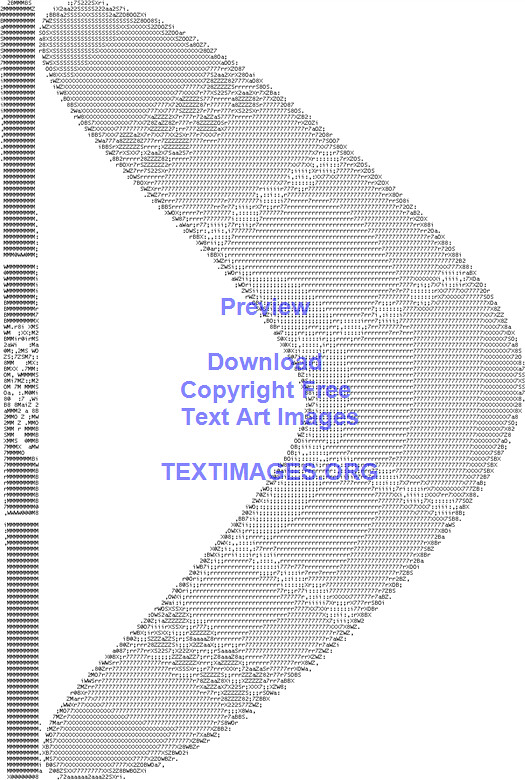The image is a detailed artist's rendering primarily featuring a gray boomerang adorned with lighter and darker gray circles in an alternating pattern. The boomerang is centrally positioned and lays flat against a white background. On the left side of the boomerang, there is a round, black and white striped pole with a white symbol at its center. The boomerang appears to be attached to this pole, with both ends of the boomerang making contact with it. 

Above the boomerang, there is text in purple that reads, in descending order: "Preview," "Download," "Copyright free text art images," followed by the website "textimages.org." The boomerang and pole are created using text art techniques, adding a unique schematic quality to the image. There are no other objects in the background, making the detailed artistic elements of the boomerang and pole the primary focus of the image.